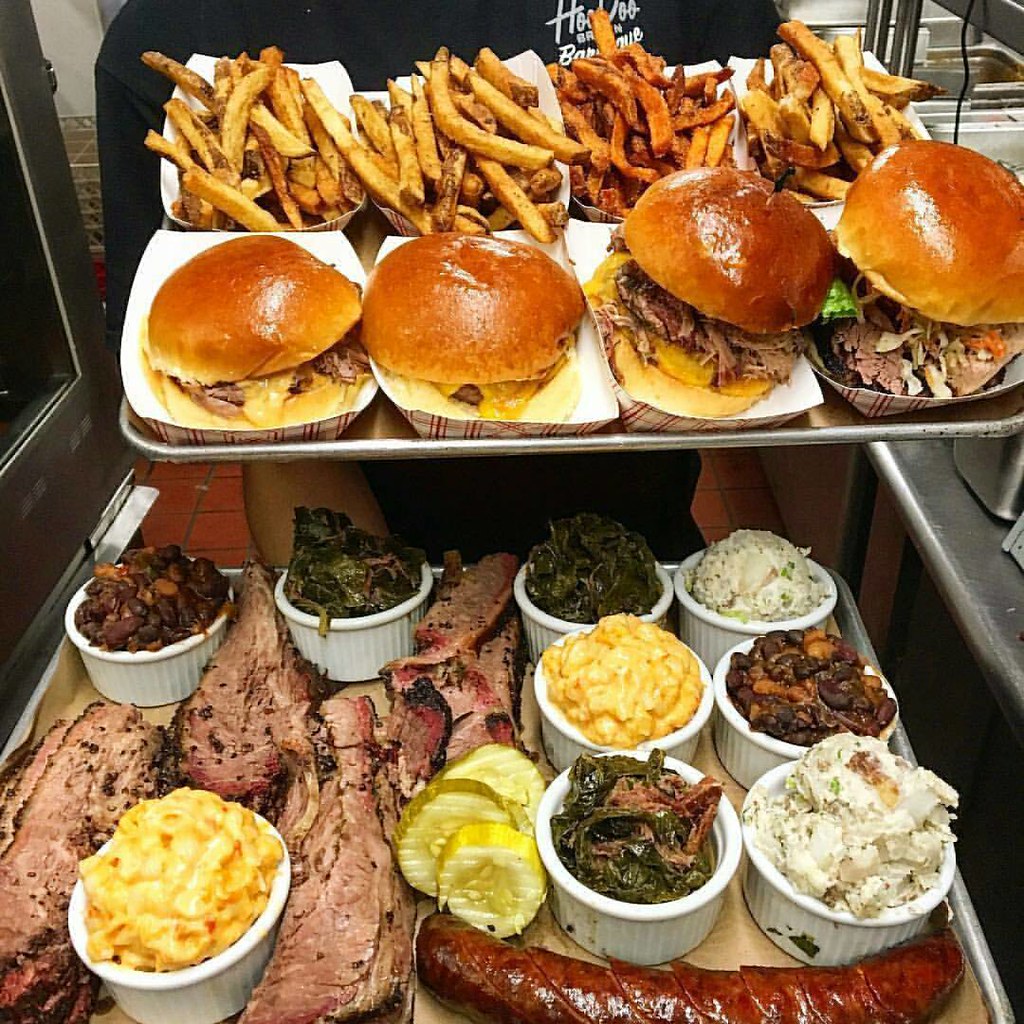The image depicts a person, whose torso is visible wearing a black t-shirt with white text, holding up two large trays of food, likely from a barbecue restaurant. The top tray, positioned higher in the image, contains four servings of French fries—one of which appears to be sweet potato fries—and four sandwiches, possibly pulled pork or barbecue sandwiches, arranged in two rows of two. The lower tray is laden with an assortment of barbecued meats including slabs of brisket and a large, sliced sausage. Additionally, this tray boasts a variety of sides: mashed potatoes, baked beans, mac and cheese, collard greens, coleslaw, and pickles scattered in the center. The trays seem heavy and packed, suggesting a hearty feast is about to be enjoyed.